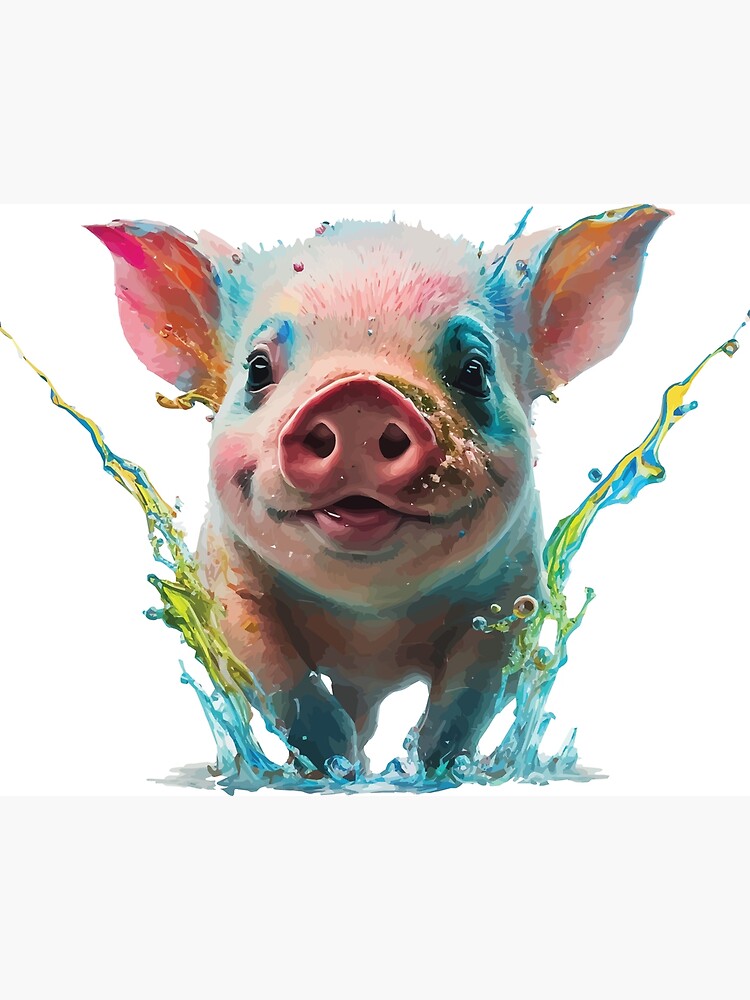This playful, AI-generated image depicts a cheerful pig joyfully splashing through vibrant water. The pig, primarily pink, features an array of colors: blue on its head and around its eyes, and yellowish hues emanating from its ears. With a big, very pink nose and expressive black eyes, the pig exudes happiness. Water, initially blue, splashes up in cartoonish arcs around the pig, transforming into vivid green and yellow hues. The pig's three visible legs, one of its back legs hidden behind the foreleg, reinforce a dynamic sense of movement. This exuberant scene captures a not-quite piglet, not-yet adult pig, having a delightful time, with water droplets scattered around, reflecting a spectrum of turquoise and greenish-yellow shades.